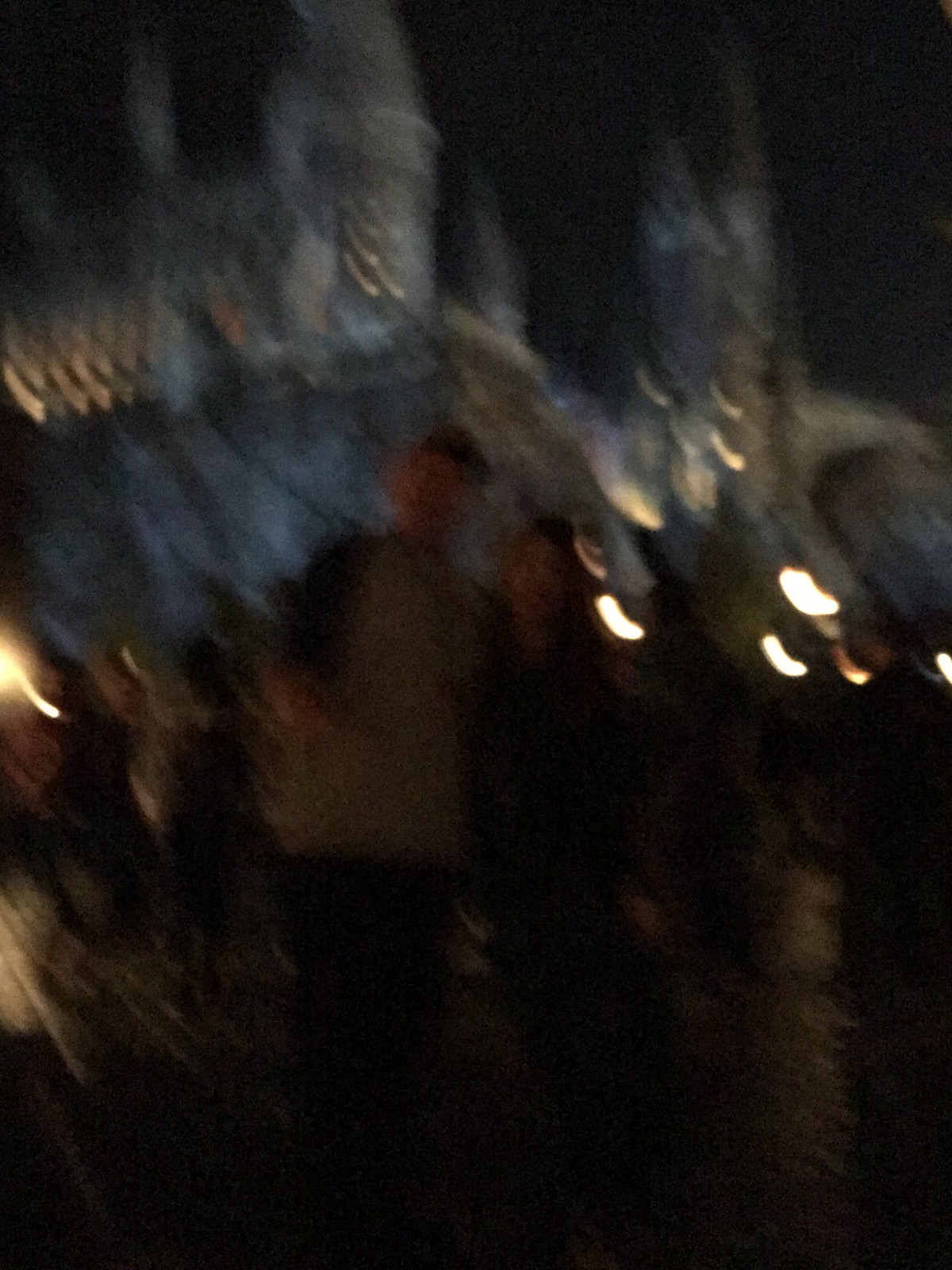This nighttime photograph features a highly blurred scene, likely due to camera motion, taken in front of what appears to be a castle. The image is very dark, with scattered sections of light resembling torches or outdoor lighting. In the foreground, two individuals with indistinct facial features are standing side by side, seemingly facing the camera and possibly with their arms around each other. One person is dressed in all black with brown hair, while the other is wearing black pants and a gray and black shirt, also with short brown hair. Additional people can be seen standing around them, though they are equally blurred and difficult to distinguish. The castle in the background has some internal illumination visible at the top left, adding a faint glow to the scene. Overall, the photograph captures a dynamic, yet indistinct moment amidst a dark, evocative atmosphere.